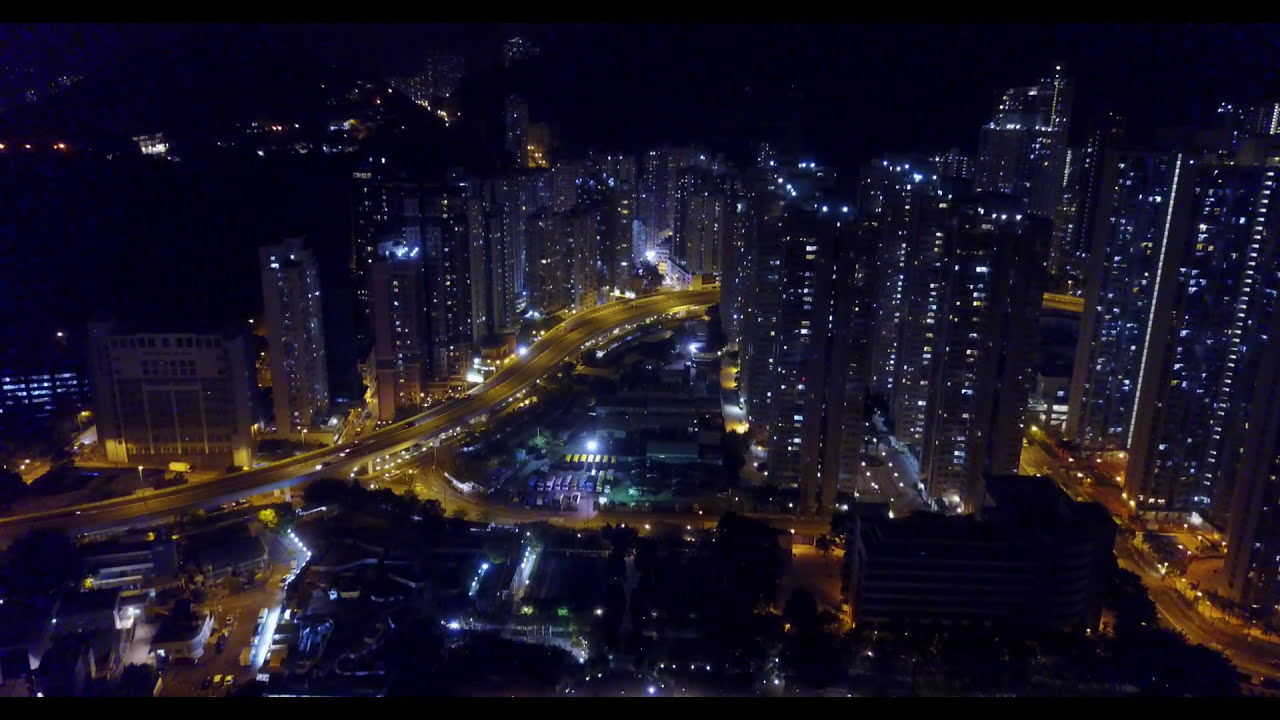This night-time photograph captures a bustling modern cityscape dominated by towering skyscrapers on both sides of a brightly lit road that extends from the left side of the image towards the center. The skyscrapers, likely residential buildings, are adorned with numerous windows emitting blue and purple lights, contrasting with the black night sky at the top of the image. At the base of these tall buildings, smaller, dimmer structures host a series of intersecting roads bathed in an amber glow from the streetlights. The scene includes multiple parking lots, with some cars parked, including a distinctive row of yellow vans equally spaced apart. The foreground is darker, showing rooftops of lower buildings, while the distant top left corner reveals another city, its presence marked by faint lights in the darkness.